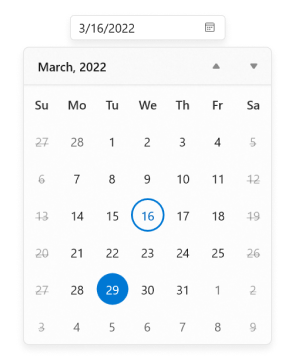This image is a screenshot of an online calendar displaying the month of March 2022. At the top of the screen, there is a search bar where "3-16-2022" is entered. Below the search bar, a vertically rectangular box shows the entire layout of the month. 

A pale gray banner across the top displays "March 2022" in black text, accompanied by up and down arrows on the far right for navigating through different months. The days of the week are listed in a row from left to right, starting with "SU" for Sunday, followed by "MO" for Monday, "TU" for Tuesday, "WE" for Wednesday, "TH" for Thursday, "FR" for Friday, and "SA" for Saturday.

The month grid begins with Tuesday, March 1st, ensuring the entire month is visible. Weekends, specifically Saturdays and Sundays, are grayed out and crossed with a line to distinguish them from the weekdays. 

Highlighting specific dates, March 16th is marked with a bright blue circle, and the number "16" is also colored bright blue to indicate it as the search result. Additionally, March 29th is similarly marked with a bright blue circle, but in this case, the number "29" within the circle is in white.